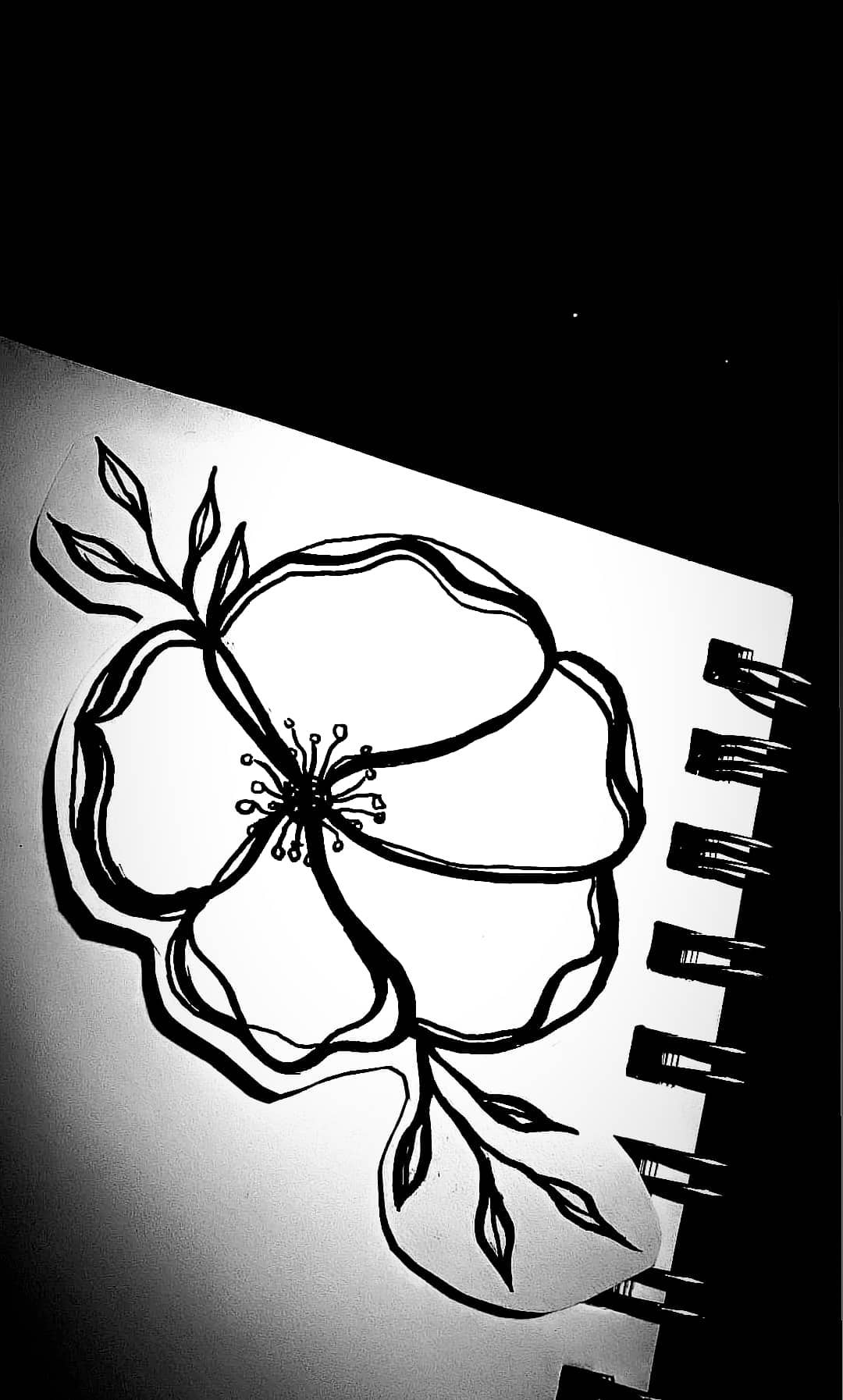This meticulously detailed black-and-white photograph captures the edge of an artist's sketchbook, bringing focus to its spiral binding visible along the right side. The entire background is engulfed in deep black, emphasizing the sketchbook fragment prominently displayed in the foreground. The upper and lower right-hand corners are completely shadowed, drawing the viewer’s attention to the intricate depiction on the sketchbook's page. The drawing, likely executed in ink, showcases a delicately rendered flower with five petals. The top and bottom of the image hint at the presence of leaves attached to the stem, while the flower's center is prominently featured, showcasing the artist’s skillful use of simple black lines to create an aesthetically pleasing piece.